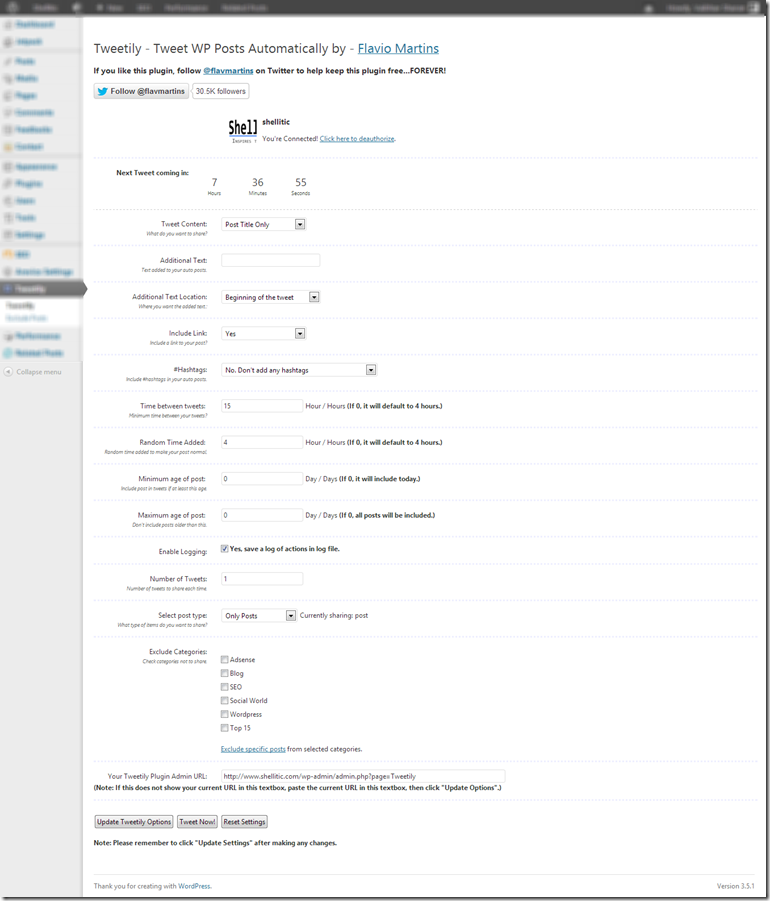This image is a detailed screenshot of a form from the Tweetily plugin interface. The background of the form is white, while other sections of the screen, including the upper left to upper right areas and the side menu from the upper left to lower left, are all blurred out. 

The visible section of the form includes the header: "Tweetily – Tweet WP posts automatically," underlined with the author "Flavio Martins." A promotional message suggests following Flavio Martins on Twitter to help keep the plugin free forever. Below this, there's a Twitter follow button displaying "@FlavMartins" with 30.5 thousand followers.

Underneath, it confirms the user's connection with the message, "Shell, you are connected. Click here to deauthorize." It also shows a countdown for the next tweet, "Next tweet coming in 7 hours 36 minutes and 55 seconds." 

The form settings include:
- **Tweet content:** Post title only.
- **Additional text:** (empty box).
- **Additional text location:** Beginning of the tweet.
- **Include link:** Yes.
- **Hashtags:** Don't add any hashtags.
- **Time between tweets:** 15 hours.
- **Random time added:** 4 hours.
- **Minimum age of post:** 0 days.

There's also a checked checkbox labeled "Enable logging" with the explanation, "Yes, save a log of actions in log file." The number of tweets is set to 1.

For post selection:
- **Select post type:** Only posts.
- **Exclude categories:** AdSense, Blog, SEO, Social World, WordPress, Top 15.
- **Exclude specific posts from selected categories:** Options available but not detailed.

Finally, the form includes three buttons: "Update Tweetily options," "Tweet now," and "Reset settings."

At the bottom, the phrase, "Your Tweetily plugin admin URL," is displayed.